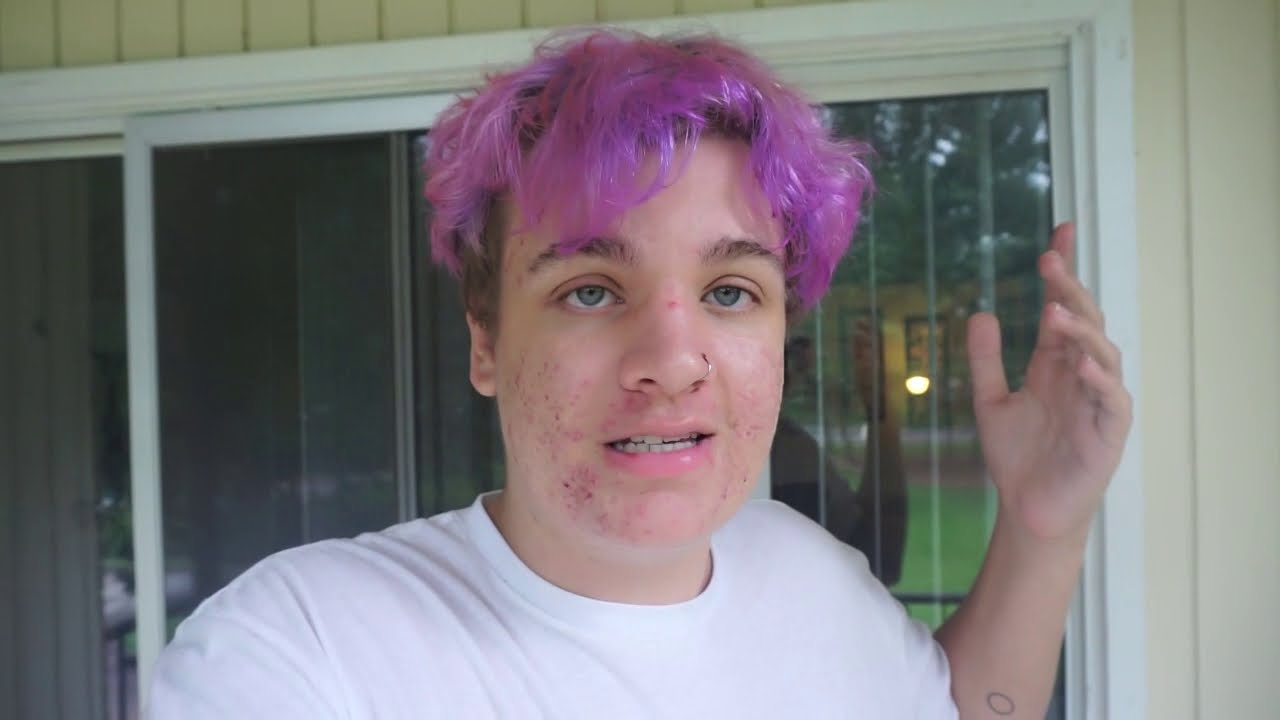The image depicts a young man, possibly in his 20s, with fair skin and striking blue eyes. He has a nose ring and noticeable acne on his cheeks. His most distinctive feature is his longish, purple-dyed hair, which contrasts with the shorter hair on the sides of his head. Dressed in a white T-shirt, the man stands in natural light in front of a sliding glass door on the side of a house, framed by light tan, vertical wood paneling. His mouth is slightly open, revealing his teeth, as if caught mid-sentence, and his left hand is raised in an expressive gesture, enhancing the impression that he is in the midst of a conversation. Additionally, tattoos are visible on his skin.